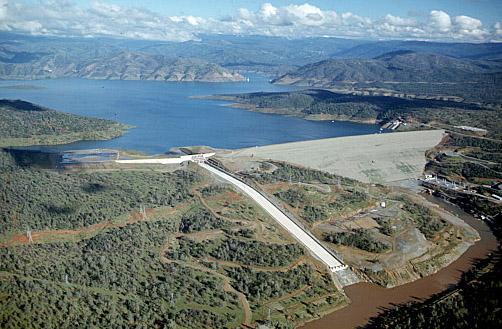This captivating real-life aerial photograph showcases a vast and impressive landscape. Occupying the upper eighth of the image, the blue sky features scattered white, fluffy clouds, creating a beautiful frame for the panorama below. Dominating the scene, a series of rugged mountain ranges stretches across the midsection, covered predominantly in green shrubbery, interspersed with various electrical towers. These mountain ranges encircle a massive, deep dark blue lake, forming a striking contrast against the surrounding greenery.

Prominently situated within the scene, a gray concrete dam holds back the substantial body of water, featuring a sluice gate on the left side. This sluice gate allows a controlled flow from the lake into a smaller, muddy river at the base of the dam. The significant height difference between the lake and the river below highlights the impressive engineering feat of the dam itself.

In closer inspection, the area around the dam is dotted with various roads, both dirt and concrete, likely used for maintenance purposes. Tiny structures near the dam suggest human presence and activity, although their details are not clearly discernible from this high vantage point. This sweeping aerial view beautifully captures the intricate interplay between natural landscapes and human infrastructure.